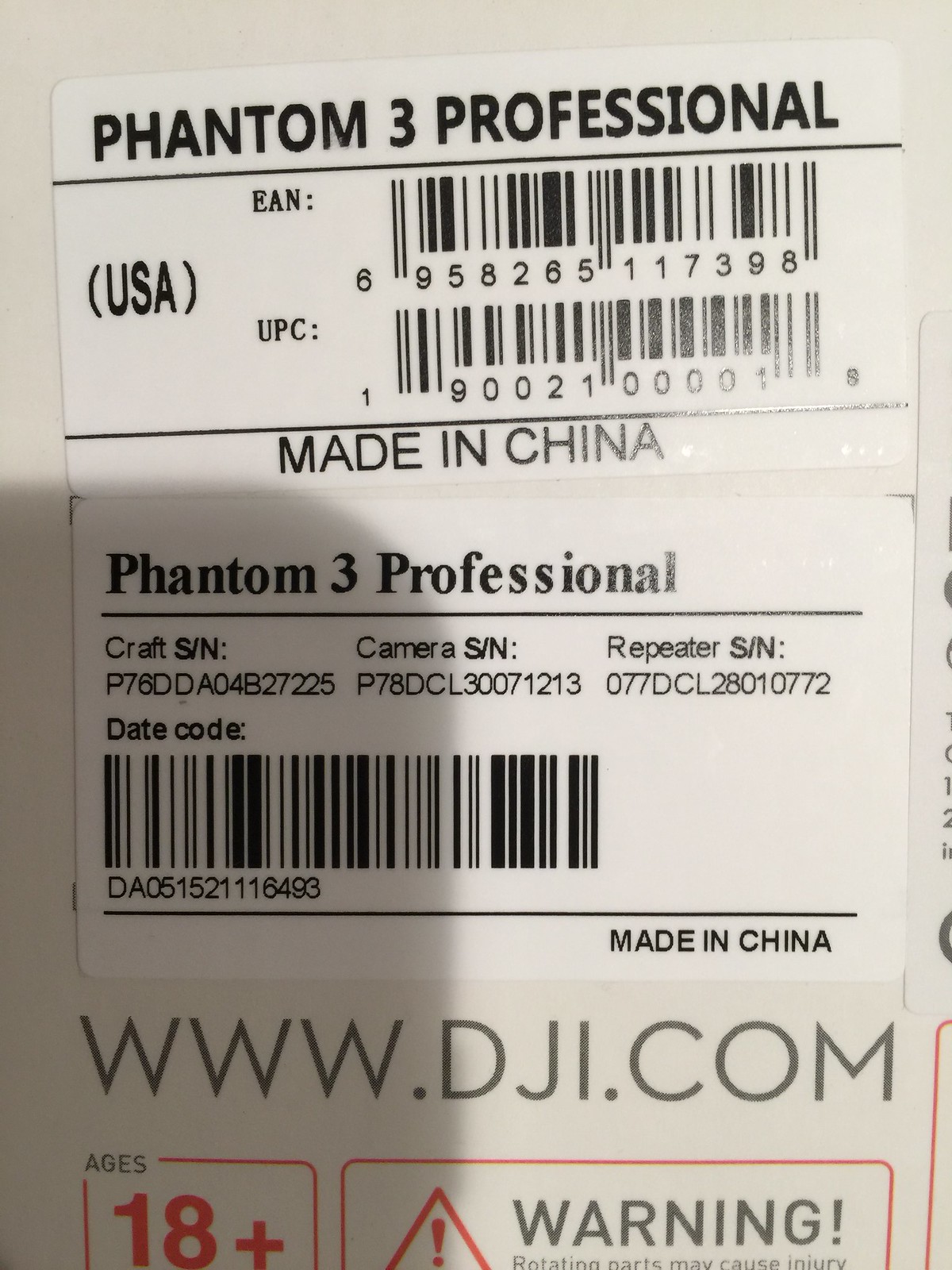The image is a detailed close-up of a label on a box, likely for a piece of equipment or a device. The top of the label displays "Phantom 3 Professional" in black text. Below this, there are mentions of "USA" and two barcodes (one possibly for Europe and another for the United States). The text "Made in China" appears more than once on the label. In the middle section, "Phantom 3 Professional" is repeated, followed by three long serial numbers labeled as Craft SN, Camera SN, and Repeater SN, which include both letters and numbers. Additionally, there is a date code accompanied by a barcode. Towards the bottom, the website "www.dji.com" is printed. There is a warning section outlined in red with an exclamation mark symbol, and text indicating that the product is for ages 18 and up, where the "18+" is prominently in red.